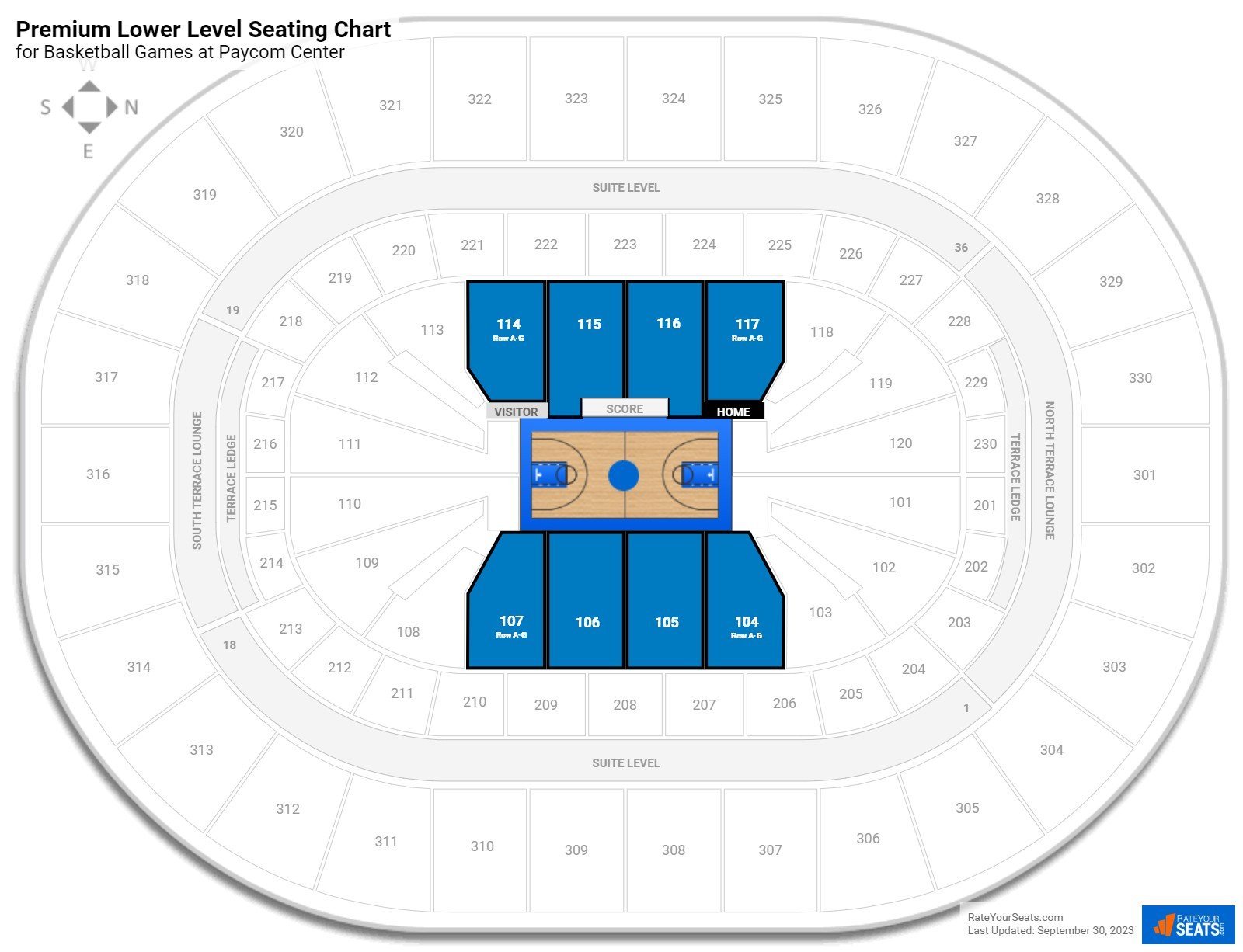This image is a detailed screenshot of the premium lower level seating chart for basketball games at the Paycom Center. The top left corner prominently displays the title "Premium Lower Level Seating Chart" in bold black letters. Just below this, in a subtler gray font, it notes that the chart is specifically for "Basketball Games at Paycom Center."

In the bottom left of the image, there is a compass with directional markers: a gray 'S' with a leftward-facing arrow, an upward-facing arrow labeled 'W' in gray at the top, a rightward-facing arrow marked 'N' in gray to the right, and a downward-facing arrow with a gray 'E' at the bottom.

Dominating the center of the image is an oval diagram representing the seating arrangement. The seating is meticulously divided into rectangular sections, each numbered for easy reference. The seating layout is composed of an outer ring and two lower tiers of seats, enveloping a centrally-located basketball court. Every detail of the seating map is precisely marked to provide an accurate representation of the premium lower level seating available for fans attending basketball games at the Paycom Center.